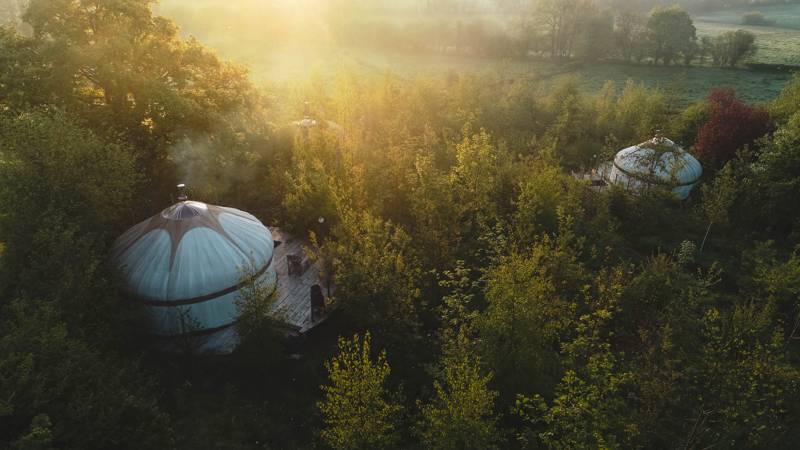The image depicts a serene, rustic area at dawn or dusk, featuring a tranquil river in the background and bathed in the golden light of the sun rising or setting from the upper left-hand corner. Taken from an aerial perspective—possibly with a drone—the scene is enveloped by a lush forest of tall, leafy green trees, with a lone tree on the right displaying striking red foliage. Nestled within this verdant grove are three elegant, dome-topped yurts, each set upon a wooden deck. Some decks have lawn chairs, and a light fog adds a mystical touch to the field beyond the grove. The yurts are positioned strategically: one in the foreground to the left, another farther down to the right, and a possible third yurt subtly visible further down to the left. The presence of moisture on the decks and the yurts contributes to the freshness and tranquility of the setting.